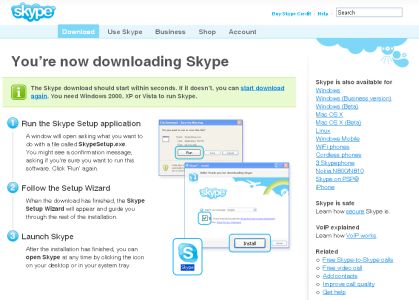The image depicts the download page of the Skype website. At the top left corner, the Skype logo is clearly displayed with white lettering and a blue outline, positioned on a white panel that spans the width of the screen. On the right side of this panel, there is a search box for user inquiries.

Directly below is a light blue navigation bar featuring various menu options such as "Download," "Skype for Business," "Shop," and "Account." The "Download" option is highlighted, indicating that the download page is currently active.

On the main part of the page, a notification states, "You are now downloading Skype." A green banner with an informational icon provides additional details about the download process, though the font is quite small and difficult to read. Below this banner, there are three sequential steps to guide users through the installation process:

1. **Run the Skype setup application**
2. **Follow the setup wizard**
3. **Launch Skype**

Each step is accompanied by a numbered blue circle and corresponding diagram.

To the far right of the image, there is an extensive list titled "Skype is also available for," containing hyperlinks to various operating systems and platforms where Skype can be used.